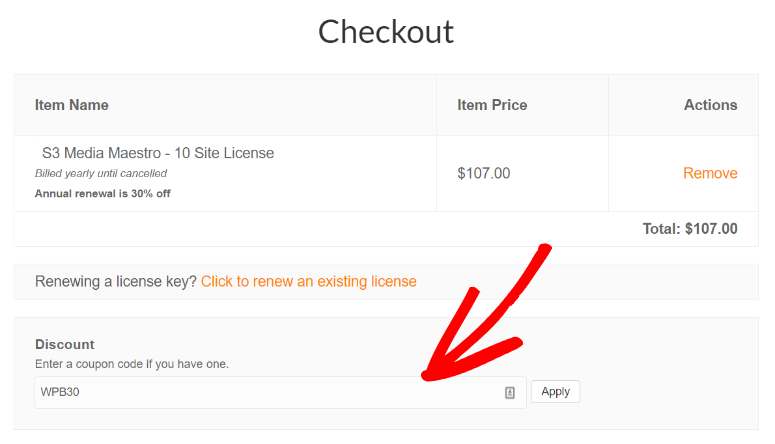The image depicts a typical online checkout page with a predominantly grey background and several highlighted sections. At the top, in bold black text, it reads "Checkout." The central focus is on an item listing for the "S3 Media Maestro, 10-site license," which is billed annually until canceled, with an annual renewal discount of 30%. The item is priced at $107. 

Below the item description, there is an "Actions" section featuring an orange "Remove" button. The total amount due is prominently displayed as $107.

Towards the bottom of the page, there is a section for renewing a license key, indicated by orange clickable text that reads, "Click here to renew an existing license."

Further down, there is a discount section where users can enter a coupon code if they have one. In this case, the coupon code "WPB30" is already entered in the provided input box. An accompanying large red arrow points to this box to draw attention to where the code should be entered. Next to the input box is an "Apply" button.

The page layout features a grey background with a few orange icons and predominantly black text, typical of online shopping checkout processes.